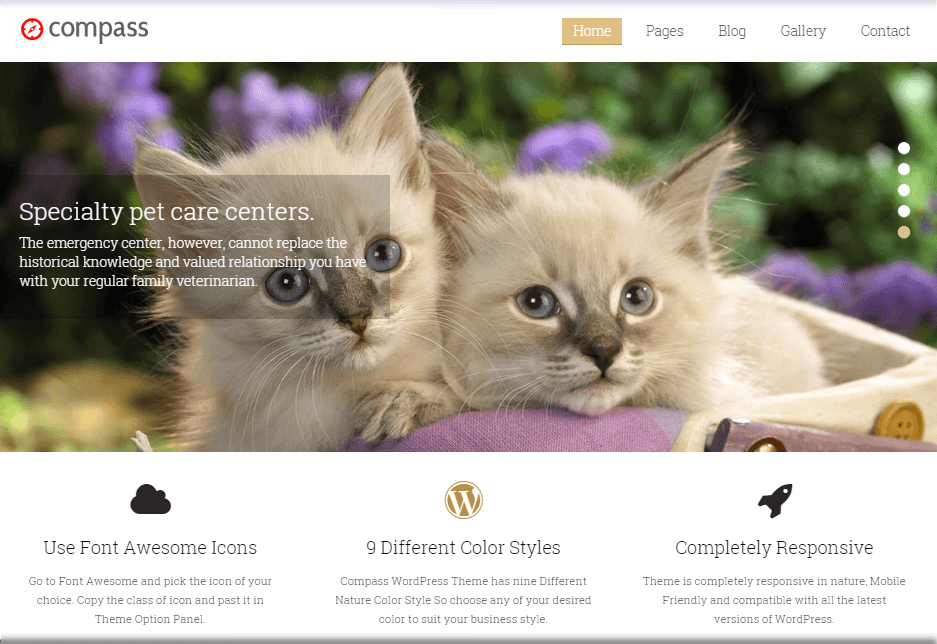This screenshot captures a webpage titled "Compass," prominently displayed on the top left along with a red compass logo. The top navigation bar, located on the upper right, includes tabs labeled Home, Pages, Blog, Gallery, Content, and Contact, with the Home tab distinctly highlighted in brown.

Dominating the top section of the page is a large banner featuring an endearing image of two beige kittens with brown noses and striking blue eyes, nestled in a purple cloth container adorned with purple flowers. The background is artfully blurred, showcasing a leafy, natural setting. To the right of this banner, a series of five dots indicate the presence of additional images, with the bottom dot highlighted, signifying the current display.

Overlaying the kitten imagery is text promoting "Specialty Pet Care Centers," accompanied by a statement emphasizing that these centers do not replace the historical knowledge and valued relationship held with regular family veterinarians.

Beneath this banner, three service highlights are presented:
1. "Use Font Awesome Icons," 
2. "Nine Different Color Styles," 
3. "Completely Responsive," each accompanied by descriptive text elucidating their features.